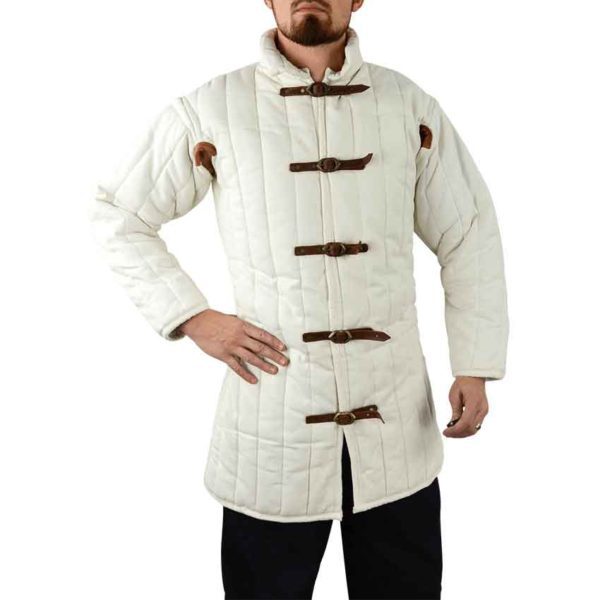The image features a man standing against a white, non-descript background, with his face visible from the tip of his nose down. He has a neatly trimmed brown beard and mustache, with visible lower parts of his ears. The man is dressed in a peculiar white or cream-colored coat that extends below his hips but not to his knees. The focal point of the coat is its unique fastening system, consisting of five short, brown leather belts instead of buttons, which run up the front of the coat to the neck. Additionally, there are brown patches of the same leather material under his armpits. The coat has a somewhat puffy appearance, with elongated sections resembling seams that run from the shoulders to the hem, and a stand-up puffy collar. The sleeves of the coat are also puffy and not tight-fitting. The man has his right hand on his hip, while his left hand hangs slightly away from his body. He is wearing black pants, visible only to mid-thigh.